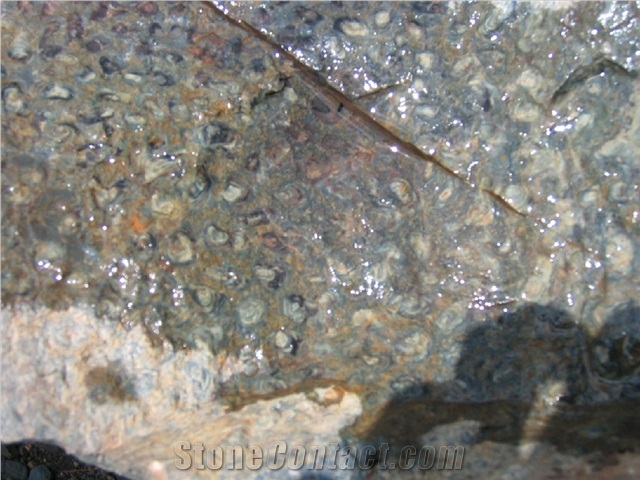This is an outdoor shot featuring a shallow, glistening water pond or lake. The water is clear enough to reveal a variety of colorful pebbles and embedded stones in shades of gray, beige, and white. Among these, there's a skinny, slippery-looking element that might be a small fish. The bottom left-hand side of the image has a lighter, whitish-gray area with some white markings, possibly a dry spot or residue on the stones. The bottom right-hand corner shows the faint shadow of the photographer. Across the bottom of the image, the words "stonecontact.com" appear in see-through, outline form, hinting that the focus might be the stones. The image quality is not very high, but it highlights the intricate textures and colors within the stone material, including a noticeable brown crack running through the middle.